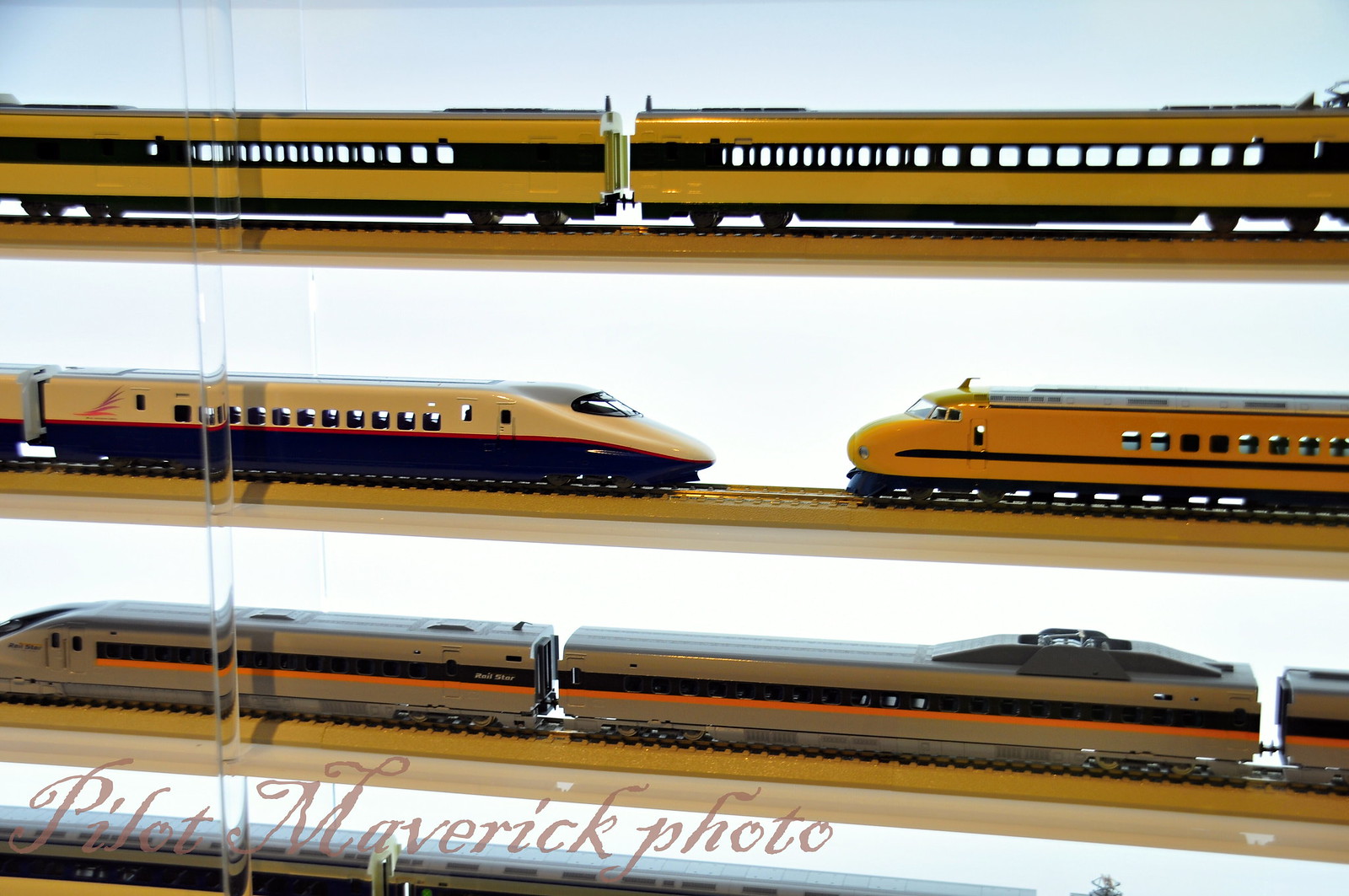The image features a detailed photograph of a multi-tiered model train set, each level showcasing different types of trains. At the bottom of the image, italicized brown text reads "Pilot Maverick Photo." The set includes three vertically stacked train tracks. 

- The topmost track displays two yellow passenger cars with black-lined windows.
- The middle track features two sleek, modern bullet trains facing each other. The left train has a silver roof, off-white sides, and a red stripe, while the one on the right is yellow with a black stripe and a gray roof.
- The bottom track has a single aerodynamic bullet train heading to the left, characterized by a gray roof and a red stripe.

The background of the image appears to be a white surface, possibly with blue undertones, suggesting a possible window or glass case behind the trains, giving an impression of an outdoor view.